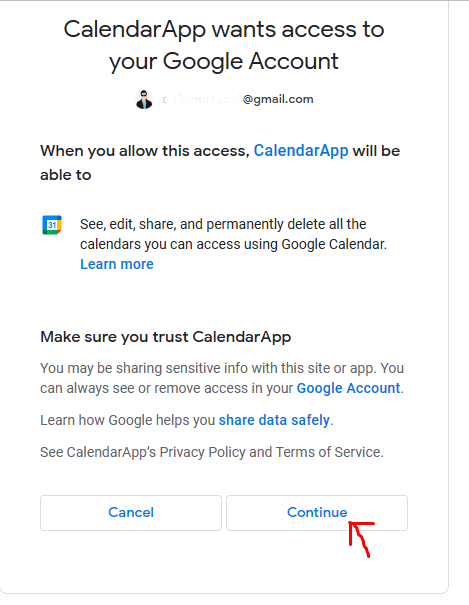This image depicts a screenshot in portrait mode with a completely white background. The focal point is a prompt requesting access for a calendar application to a user's Google account. At the top, a notification states, "Calendar app wants access to your Google account."

Underneath this notification, the user's email address is partially visible, with the username section obscured but showing the @gmail.com domain. Adjacent to the email address is the user’s avatar, although the name has been whited out for privacy.

The prompt details the permissions being requested, indicating that the calendar app will be able to "see, edit, share, and permanently delete all the calendars you use across Google Calendar." There is an advisory note encouraging the user to trust the calendar app and a warning about potentially sharing sensitive information.

Two blue hyperlinks are shown: 

1. "Learn how Google helps you share data safely."
2. "See calendar app's privacy policy and terms of service."

Interestingly, the latter is not an active link, contrary to expectations.

At the bottom of the prompt are two buttons: "Cancel" on the left and "Continue" on the right. A red hand-drawn arrow points towards the "Continue" button, emphasizing the action the screenshot's creator wants the viewer to take.